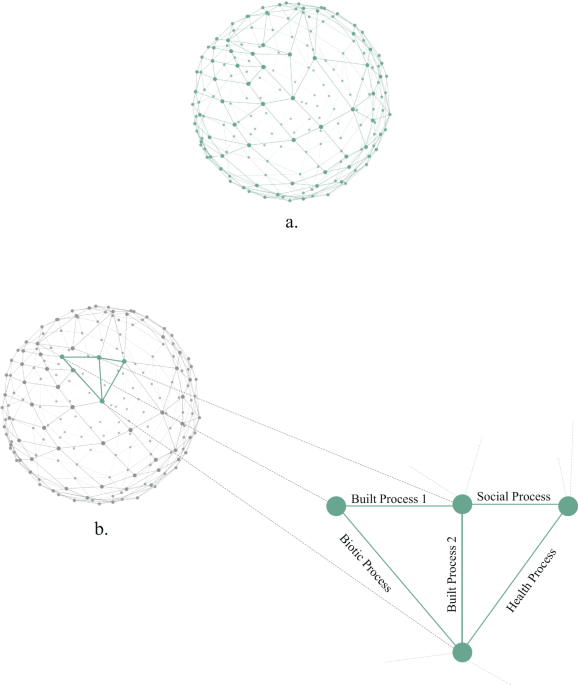The image is a detailed diagram on a white background featuring two spherical shapes, labeled A and B. Sphere A, positioned toward the top right center, is depicted with a network of green dots connected by green lines, forming a web-like structure. Sphere B, located at the bottom left, is composed primarily of grey dots and lines, with two triangular sections highlighted in green. These triangles are zoomed in on the right side of the image, displaying a more detailed view with green lines and dots. Around this zoomed-in area, black text labels various processes, including "Build Process One," "Biotic Process," "Build Process Two," "Social Process," and "Health Process." The intricate connections and highlighted regions give the diagram a futuristic and technologically advanced appearance.